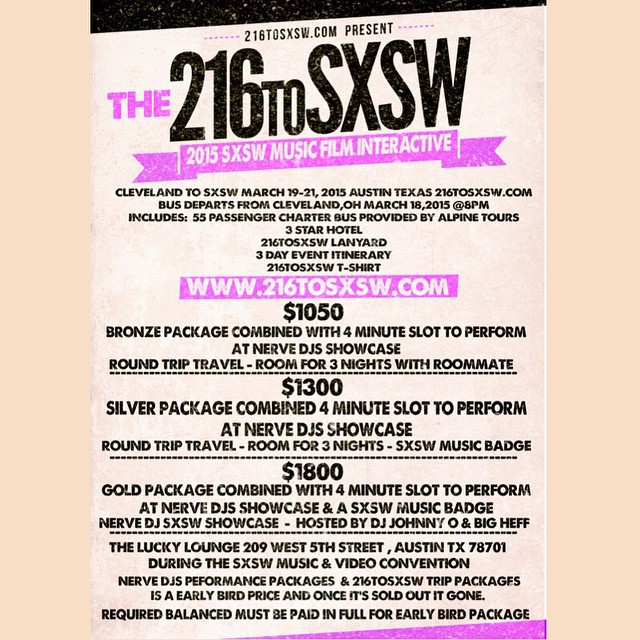This is an advertisement flyer for the 216 to South by Southwest (SXSW) Music, Film, and Interactive Festival held in 2015. The flyer has an off-white, almost eggshell yellow background, accented with large, bold black text and eye-catching pink highlights. The top prominently features the event name and website “www.216tosxsw.com,” with the words "216" and "to" in black, "the" in solid pink, and the entire URL encapsulated in a pink highlighter box. Beneath the event title, a pink ribbon banner reads "2015 South by Southwest Music Film Interactive" in white text.

The flyer details an organized trip from Cleveland, Ohio, to Austin, Texas, for the festival taking place from March 19th to 21st, 2015. The bus departs Cleveland on March 18th at 8 p.m. Included in the package are a 55-passenger charter bus provided by Alpine Tours, accommodations in a three-star hotel, a lanyard, a detailed three-day itinerary, and a t-shirt. Various packages are offered, ranging from $1,050 to $1,800, with the highest tier labeled as the "Gold Package." Additional information about pricing and packages is listed extensively on the flyer within the same consistent design theme.